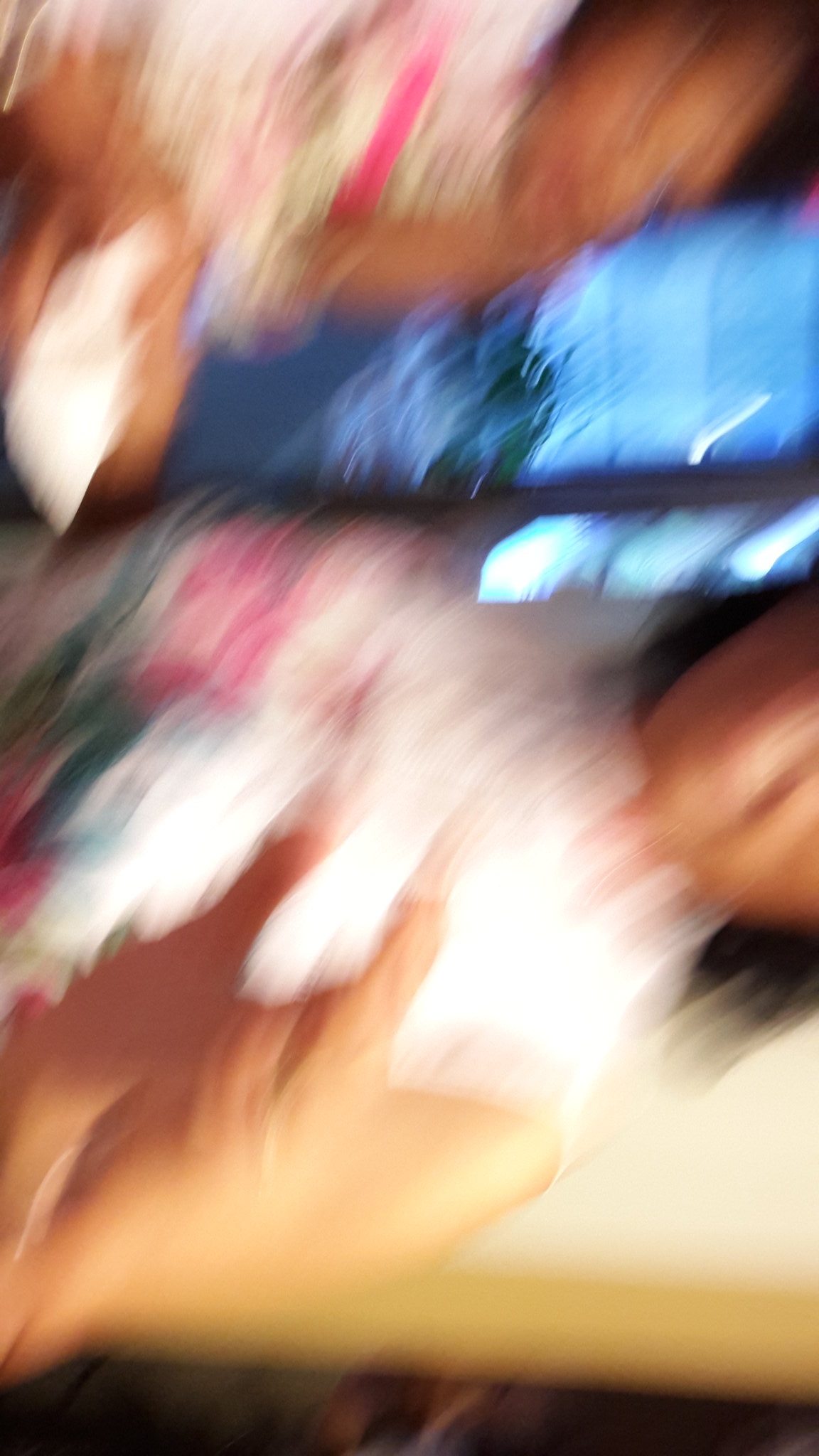This photograph, albeit very blurry and turned sideways, captures a scene involving an adult woman and a child. The woman, visibly tanned, is attired in a white dress adorned with indistinct pink and green patterns, potentially floral. Her shoulder-length brown hair frames her face, and her left hand is slightly raised. Beside her stands a child dressed similarly in a white dress with pink and green designs. The child appears to be holding its hand close to its mouth, seemingly gazing at the woman. In the background, a window reveals a blurry outdoor scene that appears to be snowy, indicated by the white patches visible through the glass.